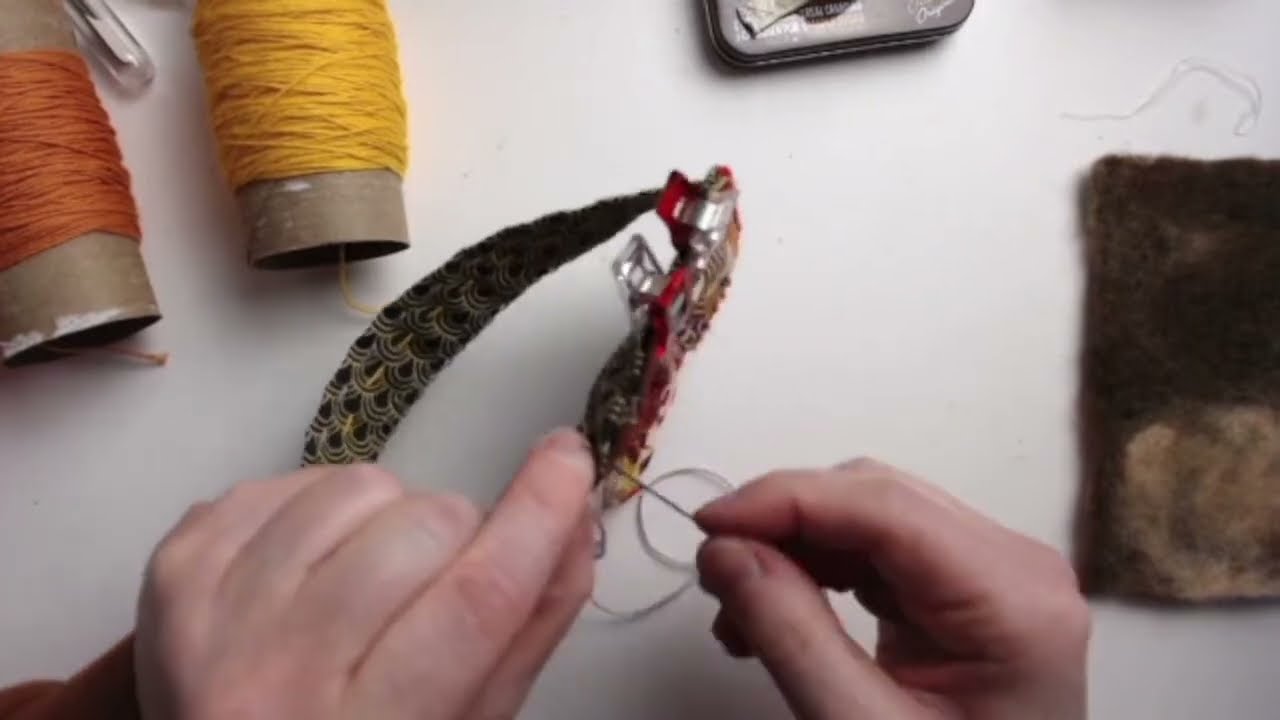In this photograph, you see a person engaged in intricately repairing a piece of beadwork, possibly adorned with gemstones. The focus is solely on their hands and the detailed beadwork, leaving their gender ambiguous. The person's hands are pale with a slight redness, and their left wrist is partially visible, indicating they are wearing a long-sleeve shirt. Their workspace consists of a white surface, which dominates the foreground of the image. 

To the left, two large spools of thick thread sit; one is yellow and the other is orange, with a cardboard tube at their cores and a transparent piece of plastic leaning against the yellow spool. On the right side, partially faded out, is a coarse, brown object that appears to be a scrubber or sponge with a rough texture. In the upper section of the photograph, a small tin or metal box can be seen, possibly a container for tools like needles. There are also clips holding the narrow band of beadwork in place as the individual works meticulously, using a needle to thread through the material.